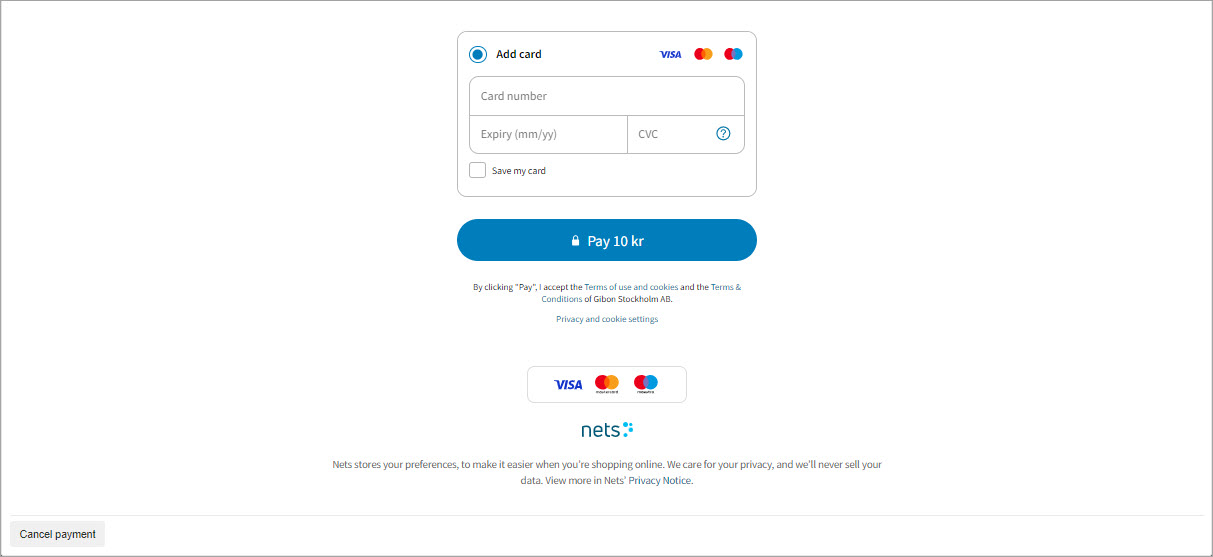The image depicts a user interface for adding a payment card, designed with a simple and clean layout. The canvas is twice as wide as it is tall and is set against a pure white background, encased within a thin black border. At the top of the image, there is a highlighted bubble that reads "Add Card".

To the right of the bubble are icons for Visa and MasterCard. Next to these is another recognizable but unidentified credit card logo, characterized by interlocking red and blue circles, similar to MasterCard's design. 

Beneath these icons is a text box labeled "Card Number", where users can input their card numbers. Directly below this, two smaller boxes are aligned side-by-side. The box on the left is labeled "Expiry (MM/YY)" for the card's expiration date, and the box on the right is labeled "CVC" for the card's security code, accompanied by a blue question mark icon for additional information.

Further down, on the left side, there is a checkbox with the option "Save my card" next to it. 

Approximately 40% down the screen and centered, a prominent blue button displays the text "Pay 10KR" in white, with a lock icon to the left, indicating a secure transaction.

At the bottom of the image are the three credit card logos again, reinforcing the accepted payment methods. Below these logos, the word "nets" is written in all lowercase letters, accompanied by a logo featuring a series of blue dots arranged in a semi-circle, pointing towards the right.